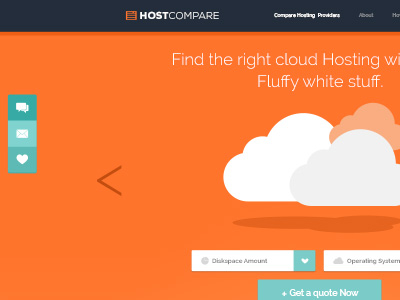This is a detailed screenshot of a webpage from a website named "Host Compared." The header of the page features a blue-gray bar that spans the top of the screen. On the left side of the header, there is an orange box displaying a logo made up of several lines. To the right of this logo, the site name "Host Compared" is prominently displayed. Further to the right, there's white text followed by two navigation links: "About" and "Home" in gray text.

The main body of the page has a vibrant orange background. Centrally positioned are vector art style cloud drawings, along with a bold left arrow. At the top of the body section, there's a prominent headline in large font stating, "Find the right cloud hosting and fluffy white stuff." Below this headline, there are two white drop-down menus, each styled as pull-down selection boxes. To the right of each white menu, there's a light blue box adorned with a heart icon.

On the left-hand side of the body section, there are three square icons in shades of blue. These icons represent a chat icon, a mail icon, and a heart icon, each housed within their respective square.

Finally, at the bottom right of the screen, a light blue box stands out with the call-to-action text, "Get a quote now."